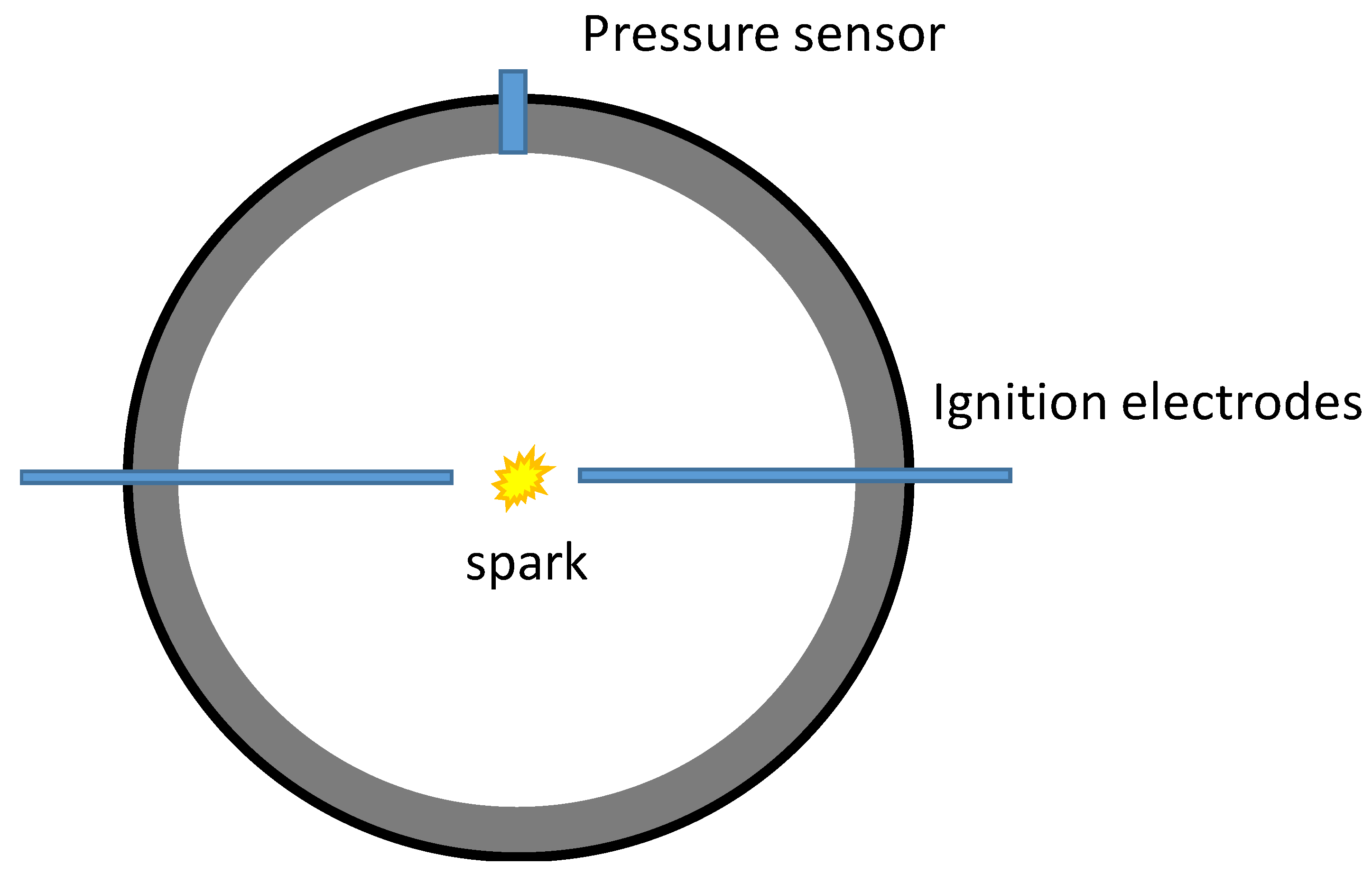This image is a detailed scientific diagram on a blank white background. It depicts a circular layout with a thin black outer border and a thicker gray inner border. At the top center, a small blue line extends from the gray border slightly past the black border and is labeled "pressure sensor" using black letters. In the very center of the white area within the circle, there is a visual representation of a spark, depicted in yellow and orange, labeled as "spark." Blue lines, representing ignition electrodes, extend horizontally from the center spark through the gray and black borders, with the term "ignition electrodes" written next to these lines. This diagram likely illustrates the working mechanism of how a spark activates various components, potentially within an electrical system or machinery, as part of an educational science resource.